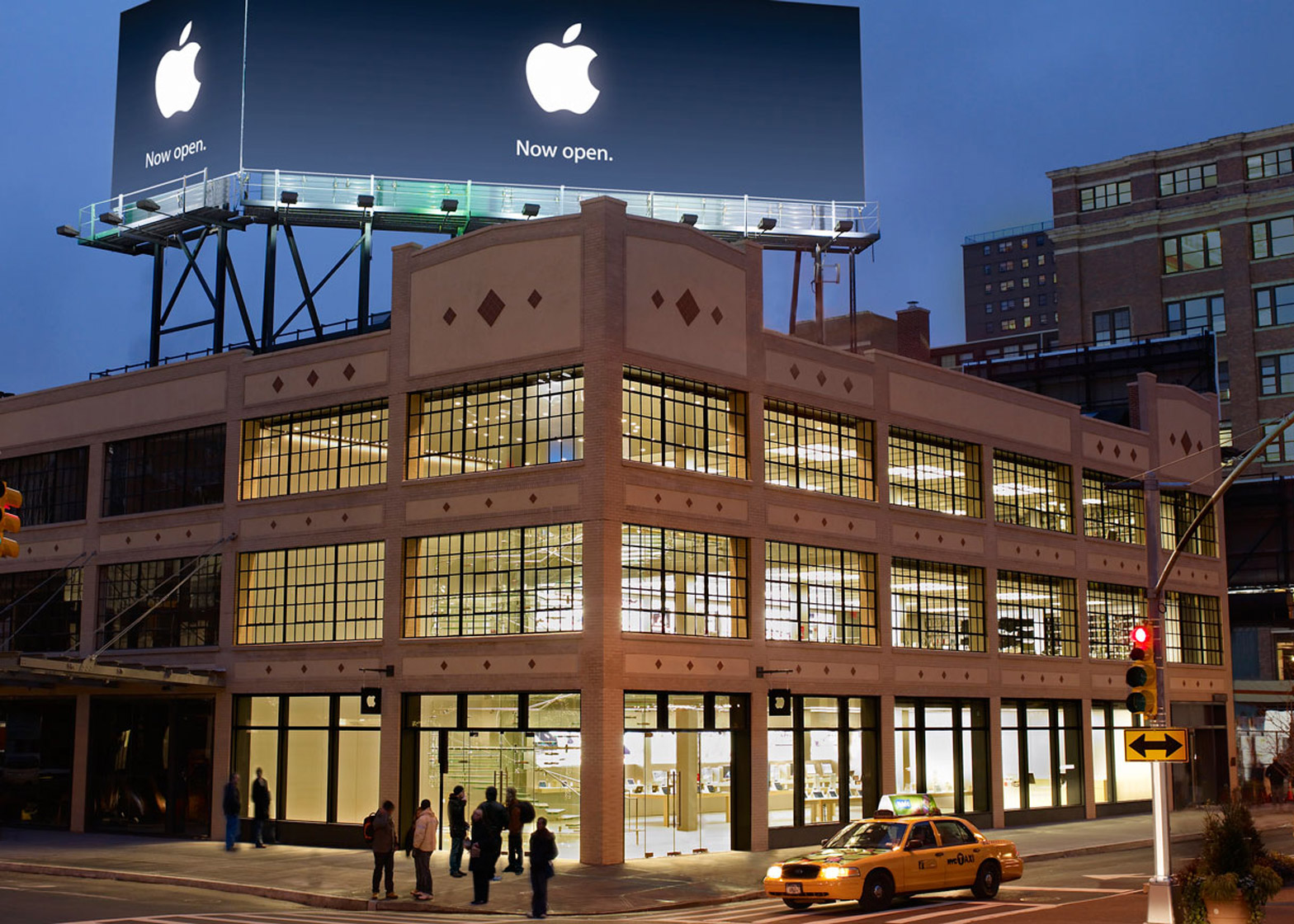In an urban setting captured at twilight or just after, the image prominently features the corner of a well-lit concrete parking garage with distinctive diamond patterns. Centered in the slightly horizontal frame, the garage has windows with 5 by 5 pane rectangular sections mounted vertically, with three such sections in each opening. In front of the garage, a group of about 8 or 9 people gathers, adding a lively touch to the scene. A yellow taxi cab is seen passing through the crosswalk at the intersection, illuminated by the streetlights. Positioned in the lower right corner, a stoplight shows a red light, while a nearby yellow rectangular sign features a two-handed black arrow. Atop the parking garage, a prominent billboard displays the message "Now Open" alongside the Apple logo on a blue-gray background, signaling the excitement of new business in the area.